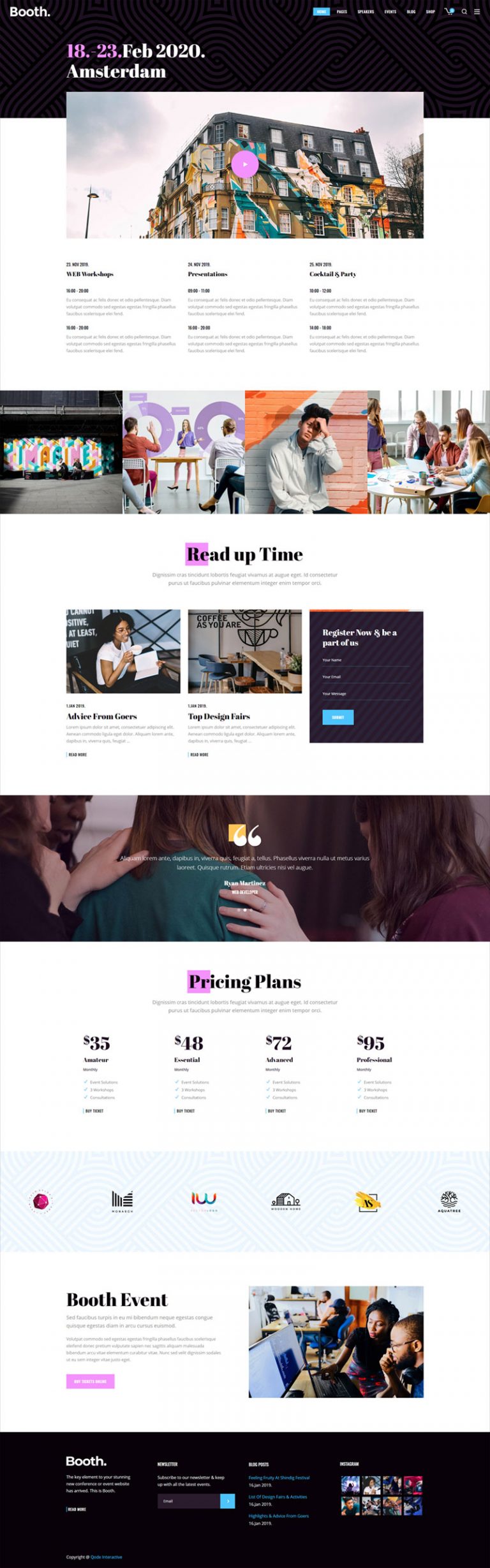In this image, we observe a well-organized event flyer or webpage detailing an upcoming event scheduled for February 18 to February 23, 2020, in Amsterdam. The content includes critical information and imagery designed to attract potential attendees. The 'Read Up Time' section likely provides a brief overview or highlights of the event.

Pricing plans are clearly outlined, catering to various attendee levels:
- Amateur: $35
- Essential: $48
- Advanced: $72
- Professional: $95

The event also promotes youth activities.

Several images enhance the flyer, depicting scenes from previous events to provide a visual context:
- A group of individuals gathered around a coffee table, focused on a laptop, suggesting collaborative work or a casual meeting.
- Participants attentively seated at a seminar, indicating educational or networking sessions.
- Someone enjoying a cup of coffee, emphasizing the social and relaxed atmosphere.
- Individuals standing in front of a monitor, possibly involved in a demonstration or discussion.

Additional text sections hint at the inclusion of a newsletter and blog posts, which likely offer further details or updates related to the event.